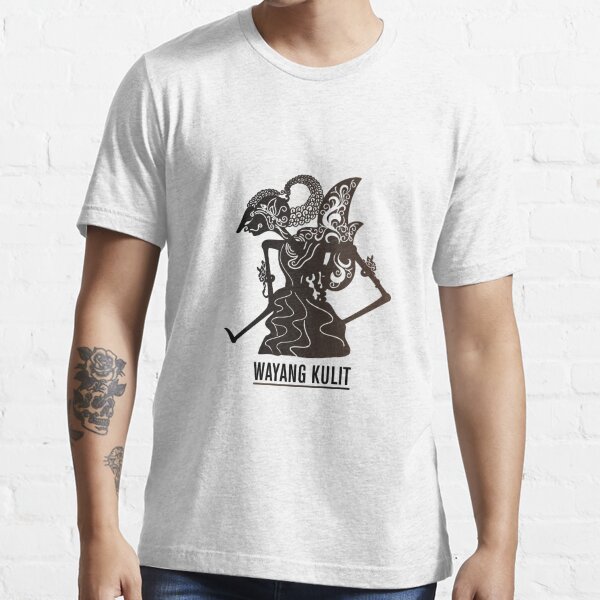The image depicts the torso of a Caucasian male wearing a white t-shirt, standing against a white brick background. The man's face and legs are not visible; only his torso, neck with a prominent Adam's apple, and arms are shown. The white t-shirt is adorned with black text that reads "WAYANG KULIT," an unfamiliar term to the observers that may reference abstract or cultural art. The artwork on the t-shirt includes an intricate, abstract pattern resembling a woman, possibly dancing, alongside an indeterminate reptile with wings. Notably, the man's right arm bears a black and white tattoo featuring a rose above a skull. His left arm appears to be free of tattoos. At the bottom of the image, the hem of the t-shirt overlaps with the top of his jeans, confirming that the man is dressed casually in a monochromatic palette.